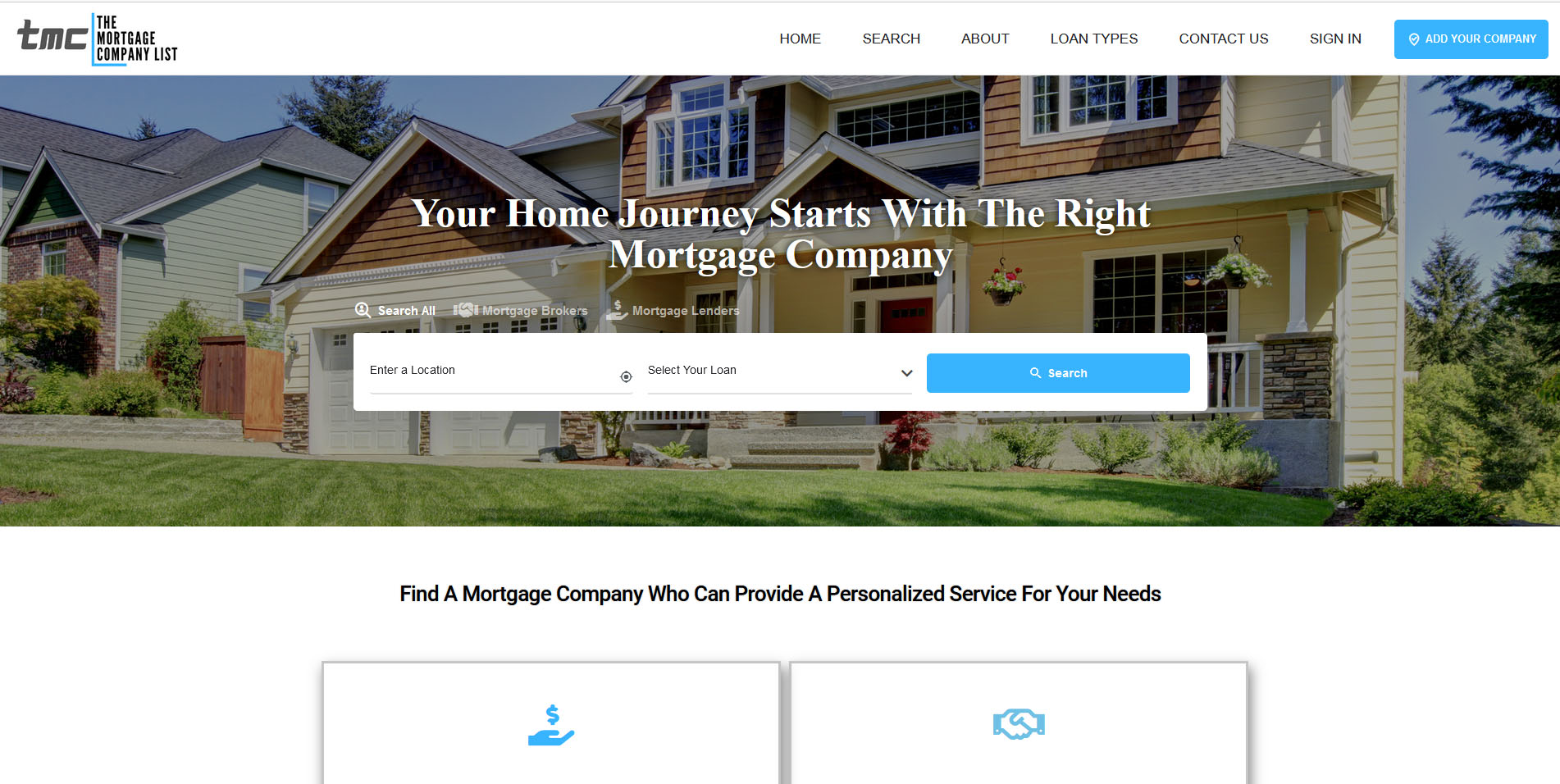This is a detailed and cleaned-up caption for the described image:

---

The screenshot appears to be taken from a computer or laptop, indicated by the format and size. At the top left, it prominently displays the title "TMC – The Mortgage Company" alongside their logo. On the top right, there are navigational menu options such as Home, Search, About, Loan Types, Contact Us, and Sign In. Adjacent to these options, a blue rectangle button features the text "Add Your Company" in white font with an accompanying symbol.

Below the navigation bar, a large banner image spans the width of the screen, showcasing a couple of homes. Superimposed on this banner are the words "Your Home Journey Starts with the Right Mortgage Company." The banner also includes options for "Mortgage Lenders," "Mortgage Brokers," and "Search All."

Directly beneath the banner, there's a search box equipped with filter options for entering a location and selecting a loan type. A small GPS icon suggests the functionality for quickly entering one's location. A blue rectangle button labeled "Search," accompanied by a magnifying glass icon, is positioned next to the search filters.

Further down, the text "Find a mortgage company who can provide personalized service for your needs" is displayed. Below this text, there is a light sky-blue image of a hand with a floating dollar sign above it. To its right, another clickable box illustrates the outlines of two hands shaking, also in the same light sky-blue color. The remainder of the image has been cropped out.